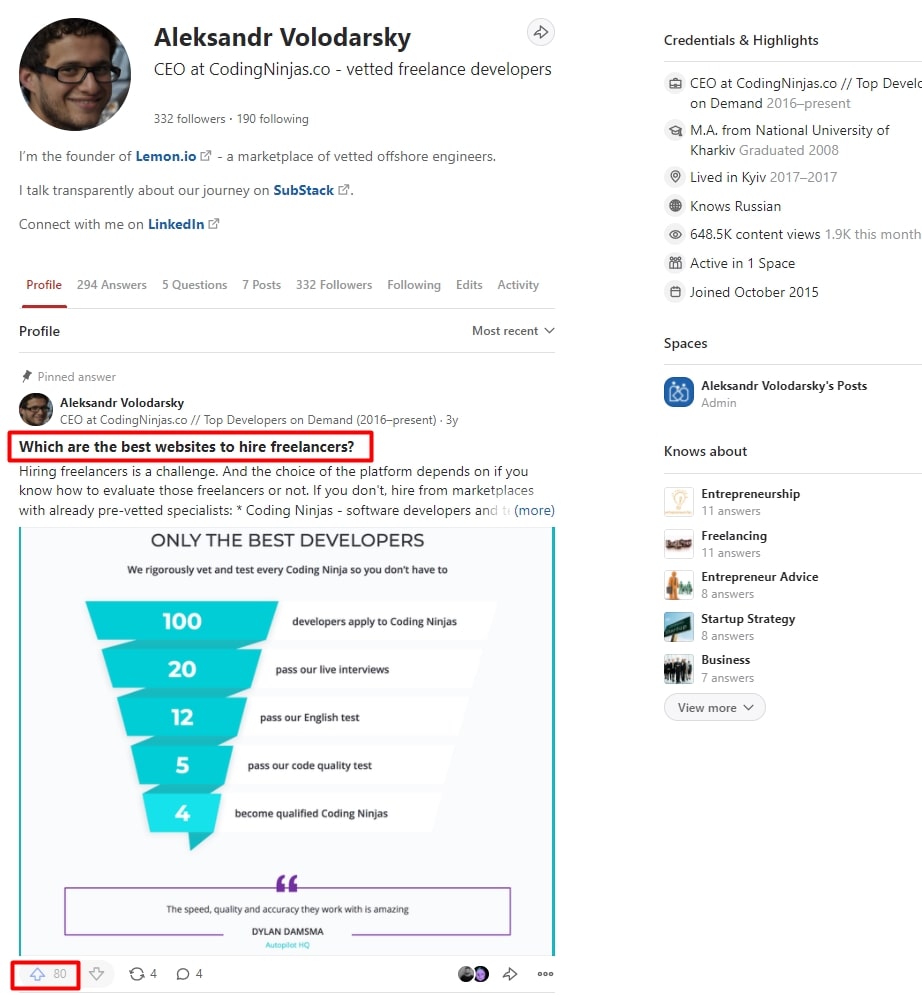**Descriptive Caption:**

This is a detailed screenshot of a LinkedIn profile belonging to Alexander Volodarsky, the CEO of CodingNinjas.co, a platform for vetted freelance developers. Alexander sports a slightly tanned complexion, curly black hair, black-framed glasses, and a bit of facial hair around his jaw and chin. He wears an engaging, albeit slightly quirky grin as he looks directly into the camera.

Alexander's LinkedIn profile proudly showcases his professional title and affiliation: "CEO at CodingNinjas.co." Impressively, he has 332 followers and follows 190 others. His profile summary reads: "I'm the founder of Lemon.io, a marketplace of vetted offshore engineers. I talk transparently about our journey on Substack. Connect with me on LinkedIn."

Below the headline, the profile interface displays a variety of selectable tabs: 294 Answers, 5 Questions, 7 Posts, 332 Followers, and Following, reflecting Alexander's activity on the platform. The profile tab is currently selected.

Pinned at the top of his posts is a highlighted question in a red text box: "Which are the best websites to hire freelancers?" Alexander's response outlines the challenges of hiring freelancers and advises choosing platforms with pre-vetted specialists, such as CodingNinjas. A clickable link provides more information.

Also featured in the screenshot is a promotional graphic captioned "Only the Best Developers." This image presents a pyramid, shaded in blue, with levels numbered 4, 5, 12, 20, and 100, symbolizing the rigorous vetting process CodingNinjas developers undergo. The pyramid's base describes the steps to become a qualified CodingNinja: passing a code quality test, English test, and live interviews.

The post concludes with a note about its popularity, indicating it has been upvoted 80 times, potentially suggesting its origin from Reddit.